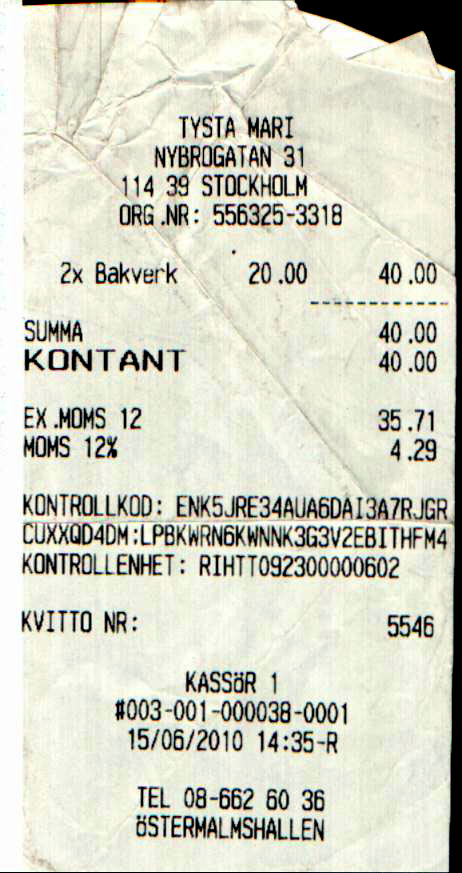This image is a close-up photograph of a crumpled and slightly dirty white receipt, suggesting it was likely carried in someone's pocket. The receipt, printed in black ink, is from a shop named "Tysta Mary," located in Stockholm, Sweden. At the top left corner, it lists the shop's address and an organization number, 556 325-3318. The receipt documents the purchase of two items, referred to as "Bakkerverk," priced at 20 each, totalling 40 in the foreign currency. Additionally, there's a tax breakdown labeled "X Moms 12" amounting to 35.71 and a corresponding tax rate, EX.MOMS12%, recorded as 4.29. At the bottom, a telephone number, 08-662-6036, is visible along with a timestamp. The receipt is surrounded by a black background that highlights its worn condition.